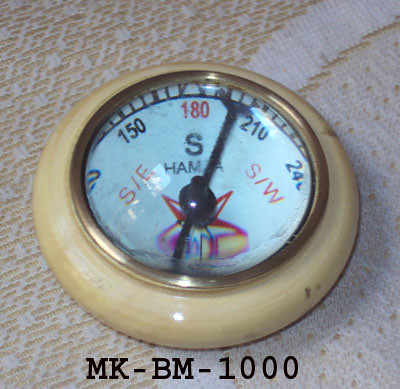The photograph showcases a compass placed directly at the center of a textured fabric background, which features a beige and white color scheme. The fabric's texture is subtly captured, adding depth to the image. The compass is composed of a light brown or beige material, with a prominent black dial. The needle points toward the upper right, indicating a direction between 180 and 210 degrees.

The compass face is clearly legible, displaying numbers such as 150, 180, and 210. The 240-degree marker is partially visible, truncated by the compass's edge. The south direction is prominently indicated with a large, black "S" at the center. To the left of it is "SE" for southeast, and to the right is "SW" for southwest, both highlighted in red. The 180-degree marker is also rendered in red, providing a strong contrasting cue.

Directly below the center of the dial, a portion of a star illustration is visible, adding a decorative touch to the instrument. Beneath the compass, the designation "MK-BM-1000" is inscribed in all caps black font, standing out against the fabric background. The detailed elements and contrasting colors of the compass are meticulously captured, providing an informative and aesthetically pleasing view.